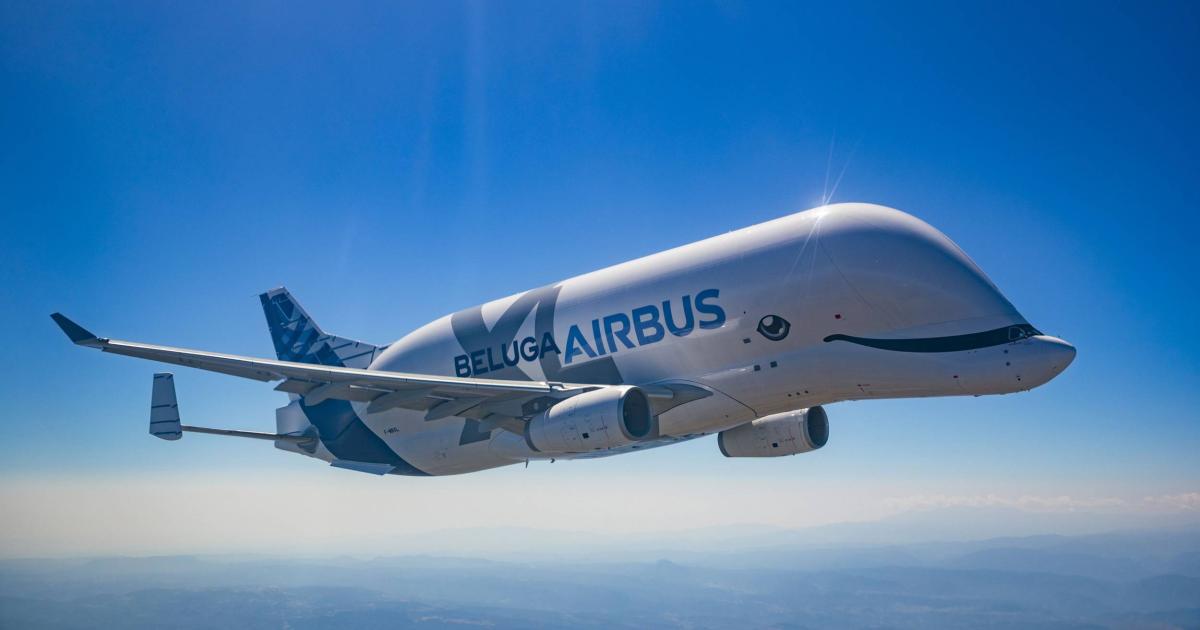In this clear and crisp aerial photograph, we see a unique airplane designed to resemble a beluga whale soaring through the bright blue sky. The Beluga Airbus stands out against a vibrant backdrop, with a gradation of blue from dark at the edges to a lighter shade toward the center, and a horizontal white cloud crossing from left to right. The aircraft itself is predominantly white, with the words "Beluga Airbus" emblazoned on its side. The front of the plane is crafted to mimic the smiling face of a beluga whale, complete with a painted eye and a slight point to its nose. The plane's tail is accented in dark blue, and two engines are visible, one on the right wing. Although a logo is present, it is difficult to discern due to its design in subtle gray lines. The overall effect is enhanced by the aircraft’s graphic wrap, making it look remarkably lifelike and whimsical.